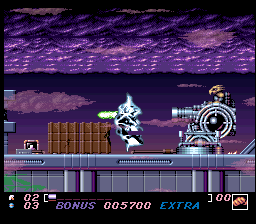This screenshot captures a moment from a retro-themed video game that exudes an ambiance reminiscent of the 1980s and 1990s arcade era. The scene is bathed in varying shades of purple, establishing a distinct color palette that enhances its nostalgic vibe. The gameplay appears to be a traditional shoot-em-up, genre recognized for its fast-paced action and vivid visuals.

In the foreground, a bird-like creature wielding a formidable cannon gun takes center stage, engaged in an intense battle. Opposing this avian warrior is a sleek, futuristic robotic character clad in a pristine white exterior, launching lightning bolts as its primary attack. The background is composed of a series of brown crates, adding an industrial touch, while the ground beneath the combatants is designed with a grid of gray cubes.

At the bottom of the screen, the word "BONUS" is prominently displayed, accompanied by the numbers "005700," possibly indicating the player's score or an in-game reward. Adjacent to this, a life indicator is visible, showcasing a collection of minuscule symbols; however, their details are indistinguishable due to their diminutive size. The overall scene intricately combines elements of classic arcade design with a vibrant color scheme, creating an engaging and visually appealing gaming experience.